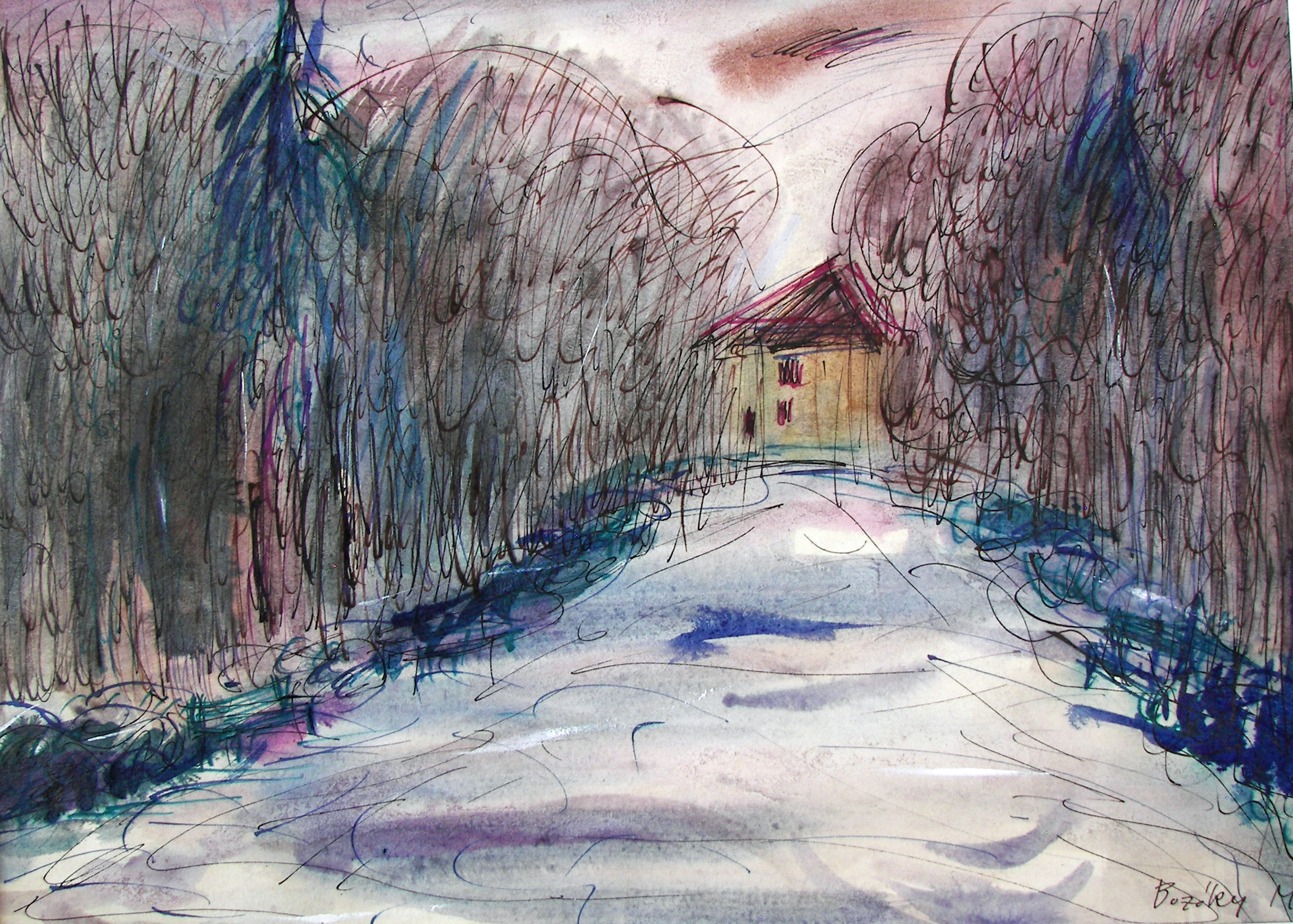This artwork is a mixed-media painting, primarily done with pencil, watercolors, and possibly oil-based paints. The scene depicts a wintery outdoor setting, characterized by a snow-covered trail that leads towards the central focal point: a house with a tan facade and a triangular red roof, complemented by two maroon-colored windows. The scene is adorned with large, barren trees on either side of the path, their dark, charcoal, and blue hues adding depth and dimension to the winter atmosphere. The sky is subtly tinted with shades of white, pink, and brown, enhancing the cold, serene ambiance. In the bottom right-hand corner, the artist's signature is visible, though only partially legible with a 'B' as the starting letter. The overall composition, with its blend of soft colors and intricate details, captures the quiet beauty of a winter’s day.